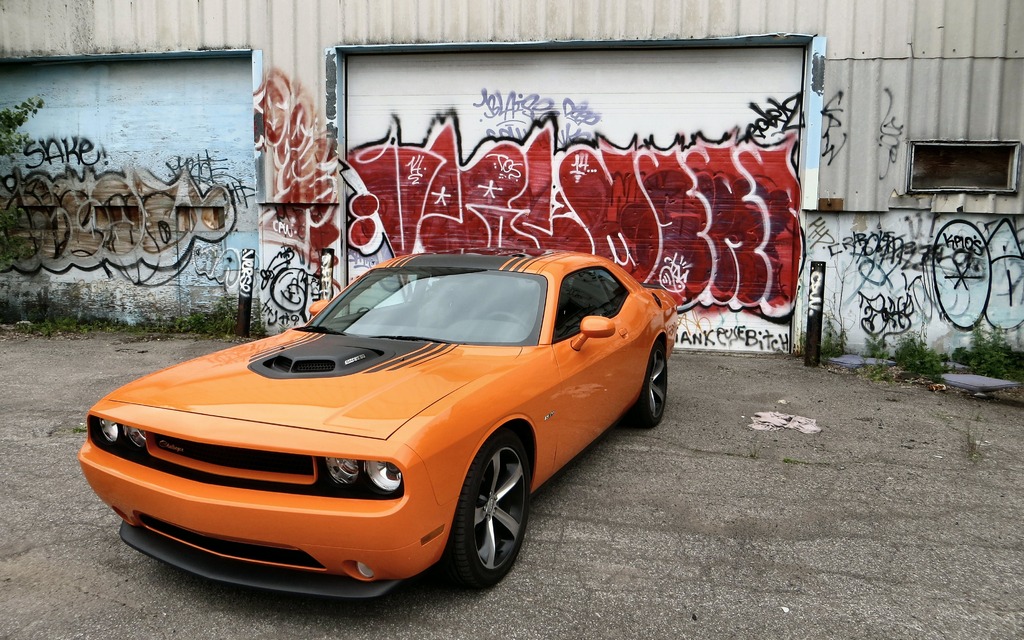The image showcases an orange muscle car, possibly a Camaro or Dodge Charger, prominently parked in front of a building with two garage doors. The car's vivid orange color is accentuated with black stripes running from the front hood, which features a raised section for an exhaust, to the roof and towards the trunk. The sleek design includes a low slung bumper under the front grille, flanked by two headlights, and the car rests on striking steel gray rims.

The building backdrop is heavily marked with graffiti. The left garage door exhibits brown graffiti with the word "sake" discernible. The central garage door, directly behind the car, is covered in red graffiti featuring large, indistinguishable letters. The adjacent building wall, adorned with more graffiti, presents a light gray vinyl siding. The car sits on a dark gray concrete ground, with patches of greenery and shrubs visible along the side of the building.